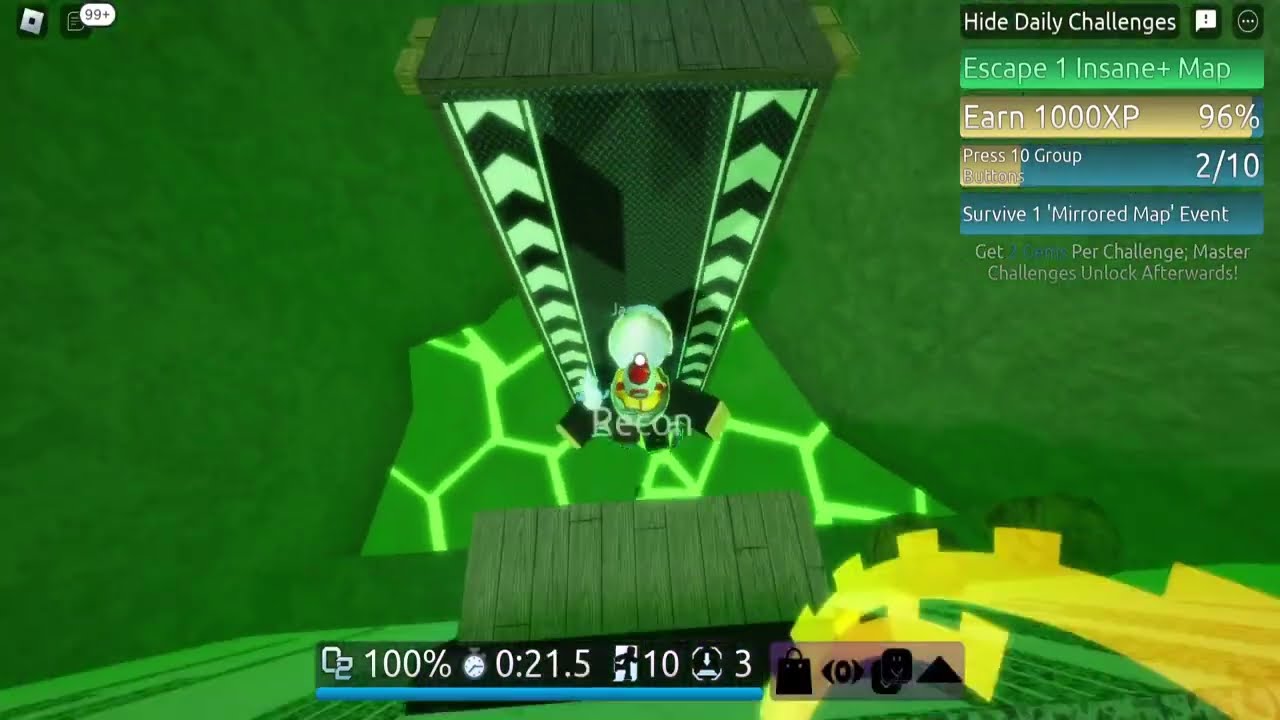The image is a screenshot from a video game displayed on a monitor or TV. The primary focus is a green grass field, possibly within a game similar to Roblox. A character with a round, white head stands out in the middle of the field, which is divided into dark green and bright green patches that appear veined. The character is situated near a black tower adorned with black and white chevron arrows pointing upward. 

In the upper right corner, there are several bars with daily challenges listed, including "Hide Daily Challenges," "Escape One Insane Map" (showing 96% completion to earn 1000 XP), "Press 10, Group, 2 out of 10," and "Survive One Mirrored Map Event." There are also notes stating "Get Per Challenge" and "Master Challenges Unlock Afterwards."

At the bottom of the screen, a blue bar indicates 100% completion. Various numbers are scattered around, such as 0.21, 0.5, 10, and 3, likely representing game statistics or progress. Additionally, a clock logo displays 21.5 seconds, and a yellow circle is present in the lower right corner. The background features a simplistic green grass landscape with a bridge.